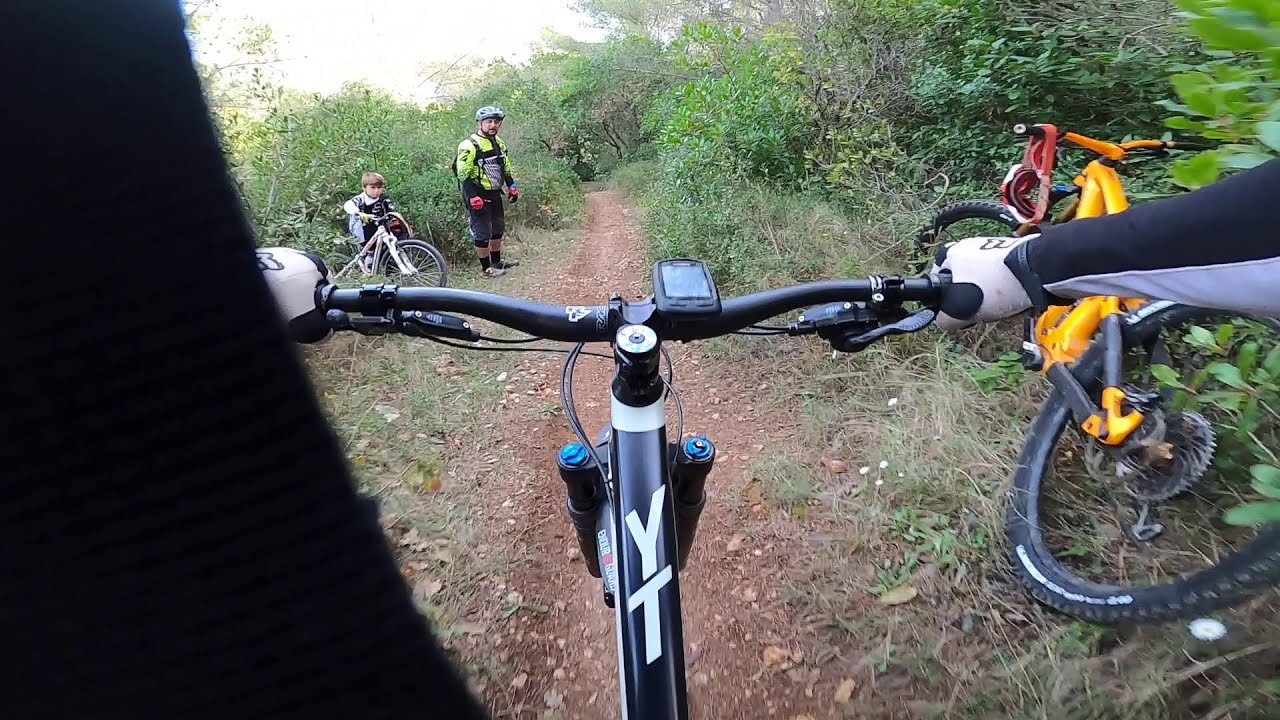In this first-person view image, a cyclist grips the black handlebars of a YT brand mountain bike, capturing their arms on either side of the handlebars and highlighting visible brake levers and the distinctive white letters on the bike's frame. The rider is navigating a dirt BMX trail surrounded by dense brush and trees, with sunlight filtering through, casting light particularly in the upper left corner. On the right side, a yellow mountain bike rests against the foliage. To the left, a man in a neon yellow shirt, helmet, and red gloves stands, accompanied by a child also in racing attire, holding a bike and waiting near the edge of the trail. The overall scene combines elements of an outdoor nature trail and a communal biking experience, emphasizing the dirt path, the surrounding natural overgrowth, and the anticipation of the onlookers.